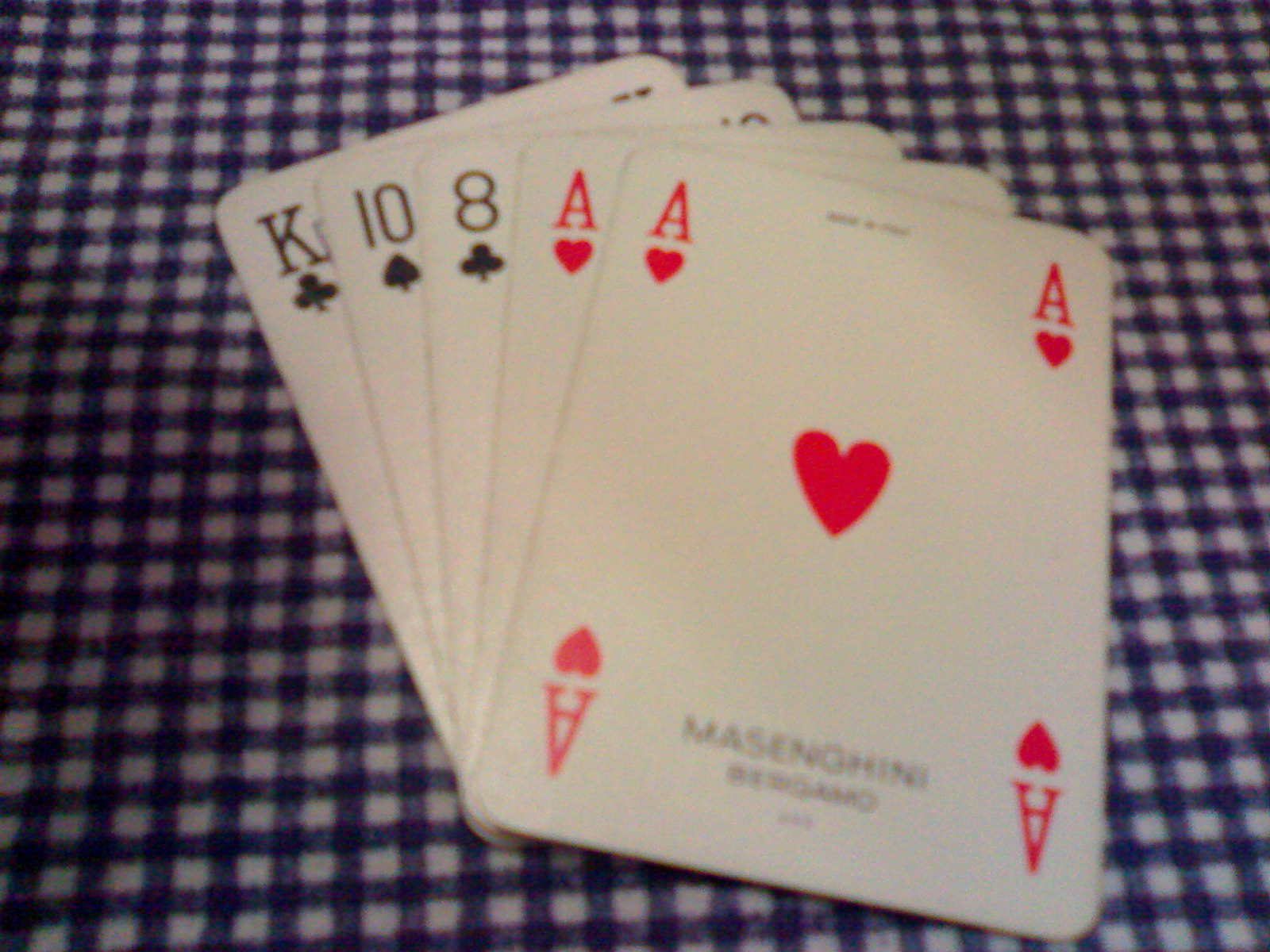The image is a close-up photograph set indoors, capturing a meticulously arranged set of five playing cards spread out on a blue and white checkered tablecloth with very small squares. Centered in the picture, the cards take up about two-thirds of the frame, with a slight darker shadow on the left-hand side. The visible cards include a red ace of hearts, another red ace of hearts, an eight of clubs, a ten of spades, and a king of clubs. The cards are neatly aligned, suggesting they were recently held in someone's hand before being placed on the table. The text "Massenghini" is visible on the cards, though slightly blurry, preventing clear reading of any additional wording below it. The overall composition and placement hint at a deliberate attempt to showcase the hand.